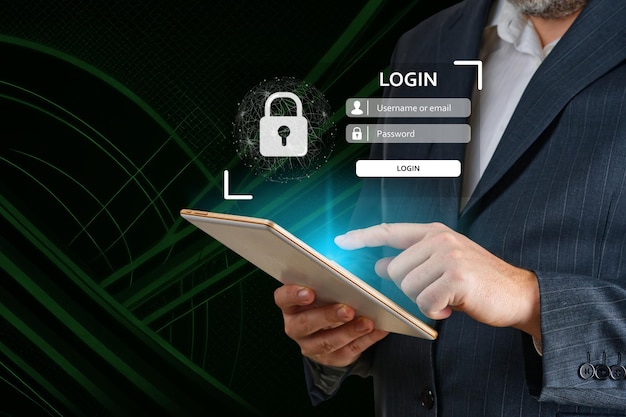The image showcases the login page of a website, featuring a geometric black background with dark green lines and shapes. At the center right, a man is depicted from the chin to the stomach area, revealing part of a gray and white beard. He is dressed in a gray pinstripe jacket with a white dress shirt underneath. The jacket's three-sleeve buttons are visible, and the jacket is buttoned up. He holds a silver tablet with his right hand while his left hand hovers over the screen, poised to interact with it, illuminated by a teal light emanating from the device.

In front of him are two key visual elements situated in the top right and bottom left corners of the image, framing a digital mesh lock graphic. The login interface is prominently displayed, featuring reversed blocks labeled "username or email" and "password," with a lock icon on the left-hand side of the password field. Below these input fields is a long, prominent "log in" button. The man's face is not shown, emphasizing the action of logging in on the tablet. The overall setting and details suggest the image could also be an ad for a secure login feature on a tablet.